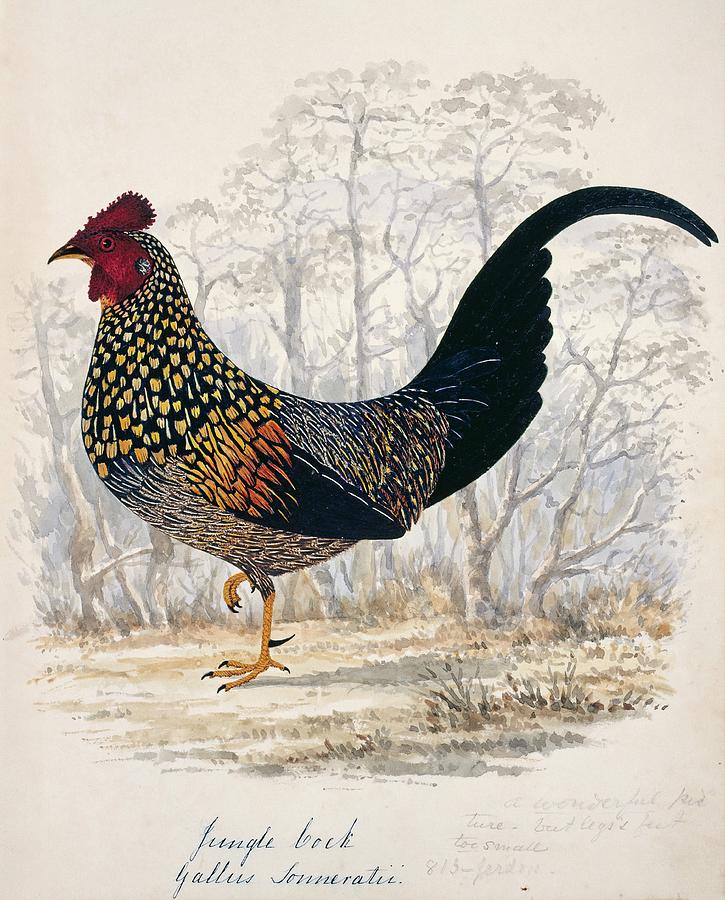The image features a detailed illustration of a rooster prominently set against a pale peach background. The rooster, rendered from a side profile facing the left, stands on its left leg with its right leg raised, showcasing a dynamic pose. The rooster’s head, strikingly red with a pronounced comb and wattles, contrasts with its black beak. Its body is adorned with black feathers speckled with yellow and orange, while its wingtips and long, curved tail feathers exhibit shades of brown. Gold-colored legs add a touch of elegance to the bird’s posture. 

The background, painted in a soft, water painting style, depicts a serene scene of forest trees in various shades of gray and light green, with patches of grass carpeting the ground. The overall color scheme is a delicate blend of pastel brown, cream, and gray tones, enhancing the tranquil ambiance of the artwork. At the bottom of the image, cursive text appears, with some parts readable as "Jungle Book," although much of it remains faded and illegible. This detailed composition, possibly meant as a piece of artwork or a greeting card, captures the essence of the rooster in a serene natural setting.